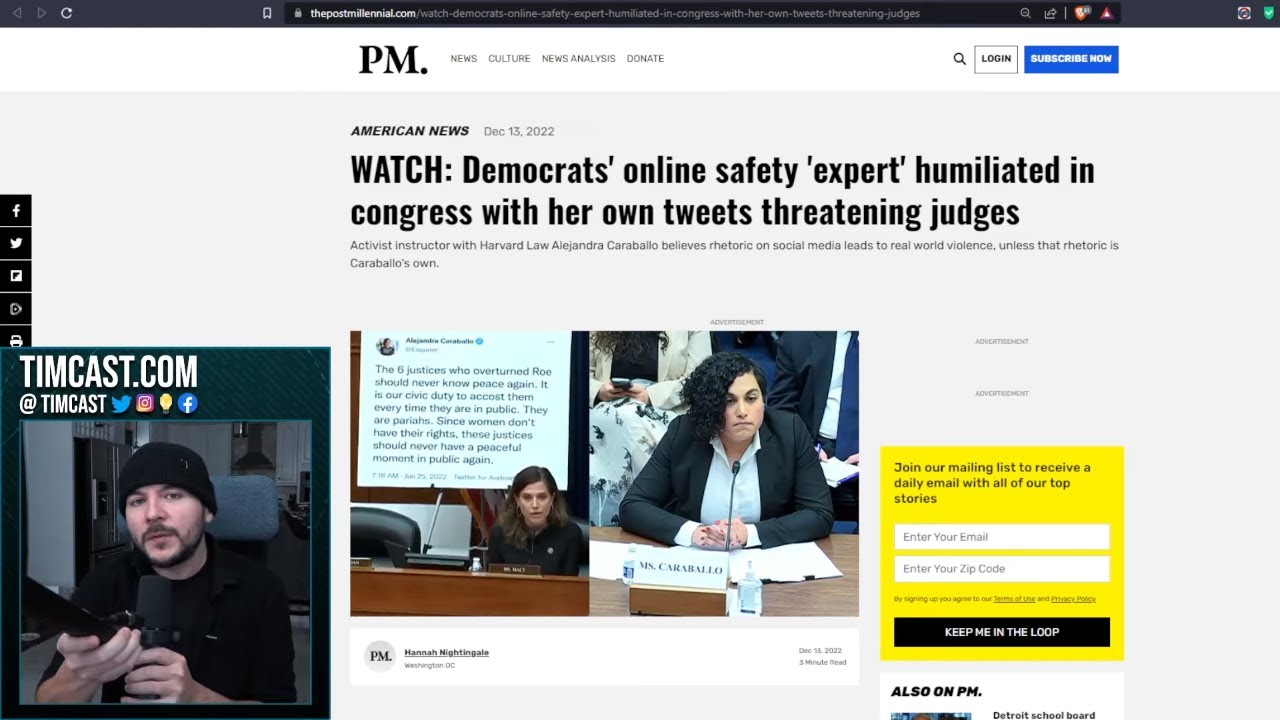This rectangular image is bordered by a thin black line along its top edge, containing small, unreadable text, a cluster of symbols on the upper left, a URL in the center, and additional symbols on the right. Directly below this border is a white banner featuring black text that reads: "PM, News, Culture, News Analyst, Donate." On the right side of this banner, there is a search function, followed by a white box outlined in gray labeled "Login," and a blue box with white text that says "Subscribe Now." The main content of the image has a gray background. Positioned at the center top are the words "American News, December 13, 2022" followed by the headline: "Watch Democrats Online Safety Expert Humiliated in Congress with Their Own Tweets Threatening Judges" in black text. Below this headline is another line of very small, hard-to-read text. The primary image also contains three embedded images overlaying it.